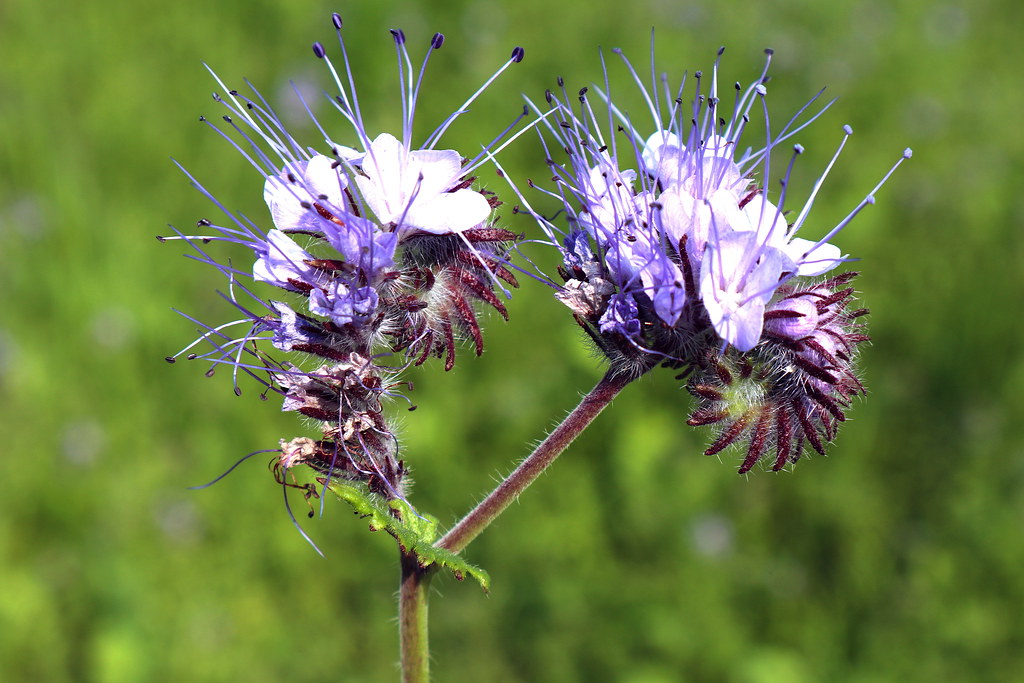This photograph captures an exquisite and unique flower with a fine level of detail. The flower features a slender green stem that bifurcates, giving rise to two distinct blossoms. Each blossom showcases a mesmerizing combination of white petals and spiky, fuzzy extensions that add to the flower's texture. Emerging from the core of each white petal are smaller stems, each ending in a delicate purple tip, reminiscent of tiny antennas. The close-up nature of the photograph highlights these intricate details, casting an almost ethereal aura on the flowers. The background, a blurred palette of greens and whites, hints subtly at its grassy nature but remains out of focus, ensuring that the vivid blossoms dominate the viewer's attention.